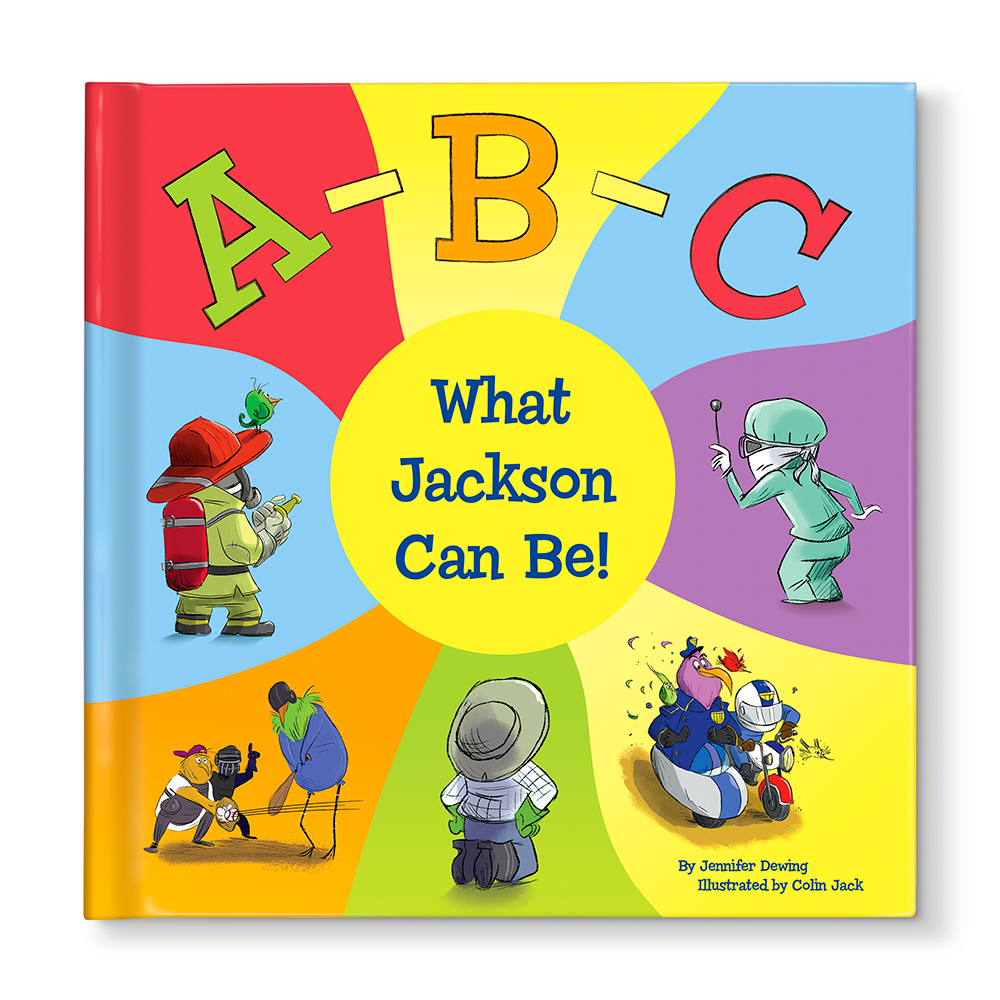The photograph is of the front cover of a children's book titled "ABC, What Jackson Can Be!" authored by Jennifer Dewing and illustrated by Colin Jack. Dominated by a multicolored pinwheel emanating from a yellow center, the vibrant, circular design instantly catches the eye. In blue lettering, centered within the yellow circle, are the words "What Jackson Can Be." Surrounding this central circle are various panels, each showcasing different professional roles that Jackson, the character, can be aspired to.

In the top-left blue segment, Jackson is depicted as a firefighter, adorned in a lime green jacket with a red hat and oxygen tank. At the seven o'clock position on a green background, Jackson appears as an umpire in a baseball scene, with two other characters—a batter, who isn't distinctly human, and a catcher catching a ball. The bottom center shows Jackson as a gardener or a farmer, dressed in a white-checkered shirt, green gloves, gray wide-brimmed hat, black boots, and jeans, kneeling and facing away from the viewer.

To the right, at the five o'clock position, on a yellow background, Jackson is shown with a football helmet, riding in the sidecar of a white-blue motorcycle, while the main rider, who has a red hubcap on the motorcycle, resembles Gonzo from The Muppets. Above this, on a purple background, Jackson is depicted as a doctor, wearing a surgical mask, cap, and gloves, and holding a small hammer, looking profession-ready.

The entire cover is festive and diverse in color and characters, providing a snapshot of various careers, illustrated in a unique, engaging style reminiscent of Dr. Seuss’s whimsy but with its distinctive charm aimed to educate and inspire children about different vocations.